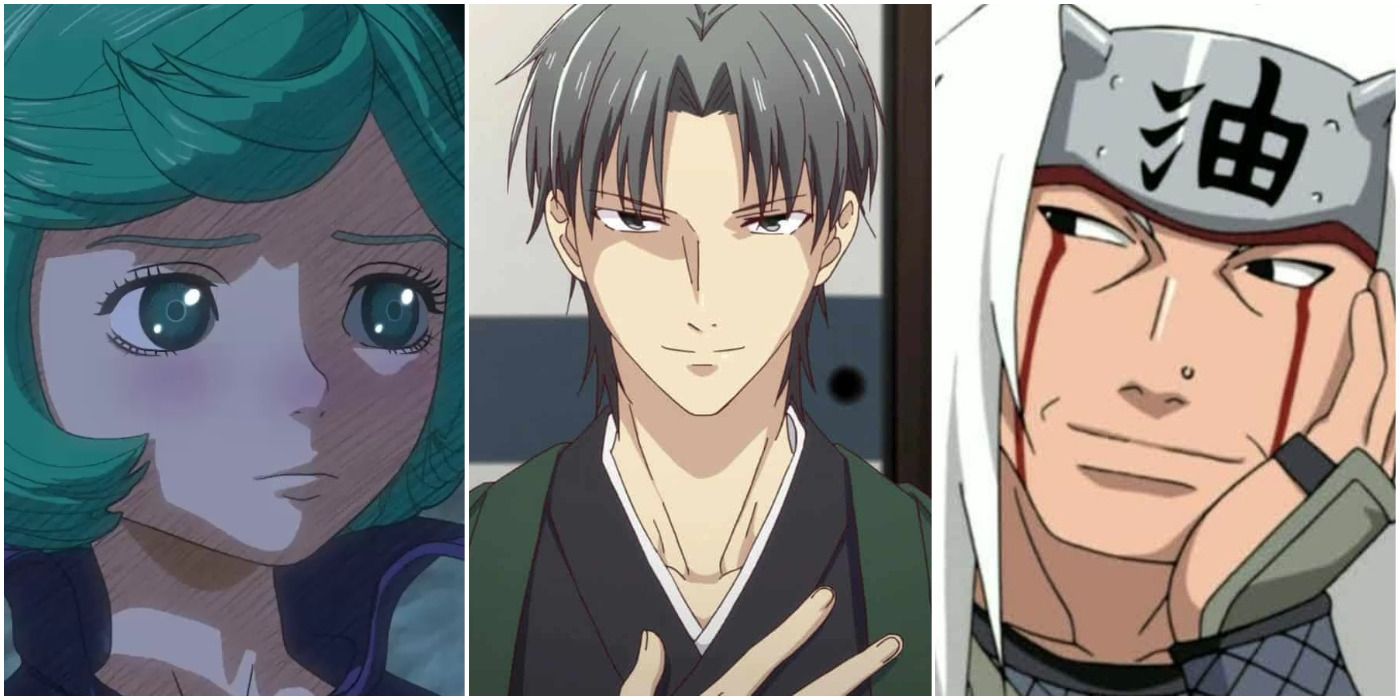This horizontally oriented image features three distinct, cartoon-esque anime-style portraits placed side-by-side. The leftmost character is a young woman with big teal eyes and short, styled, bluish-green hair featuring a wave off her bangs, complemented by teal eyebrows. She gazes solemnly to the right, exuding a sad, almost tearful expression. She wears a dark outfit with a visible high collar, possibly in shades of purple or gray. The center image showcases a young adult male with brownish-gray hair styled in bangs across his forehead. His pale eyes, which appear to be either gray or blue, look straight ahead. He is dressed in a layered outfit: a gray v-neck shirt over a white undershirt, topped with a dark green coat featuring a collar. His right hand rests over his chest. The rightmost portrait is of a man with a light complexion and Asian features, distinguished by a silver helmet adorned with Chinese symbols. He has piercing brown eyes that appear to be crying blood, with his left hand gently placed on his cheek. He wears a glove and possibly some form of silver armor, looking slightly askance. The intricate details and solemn expressions unify the trio within this digitally rendered anime artwork.